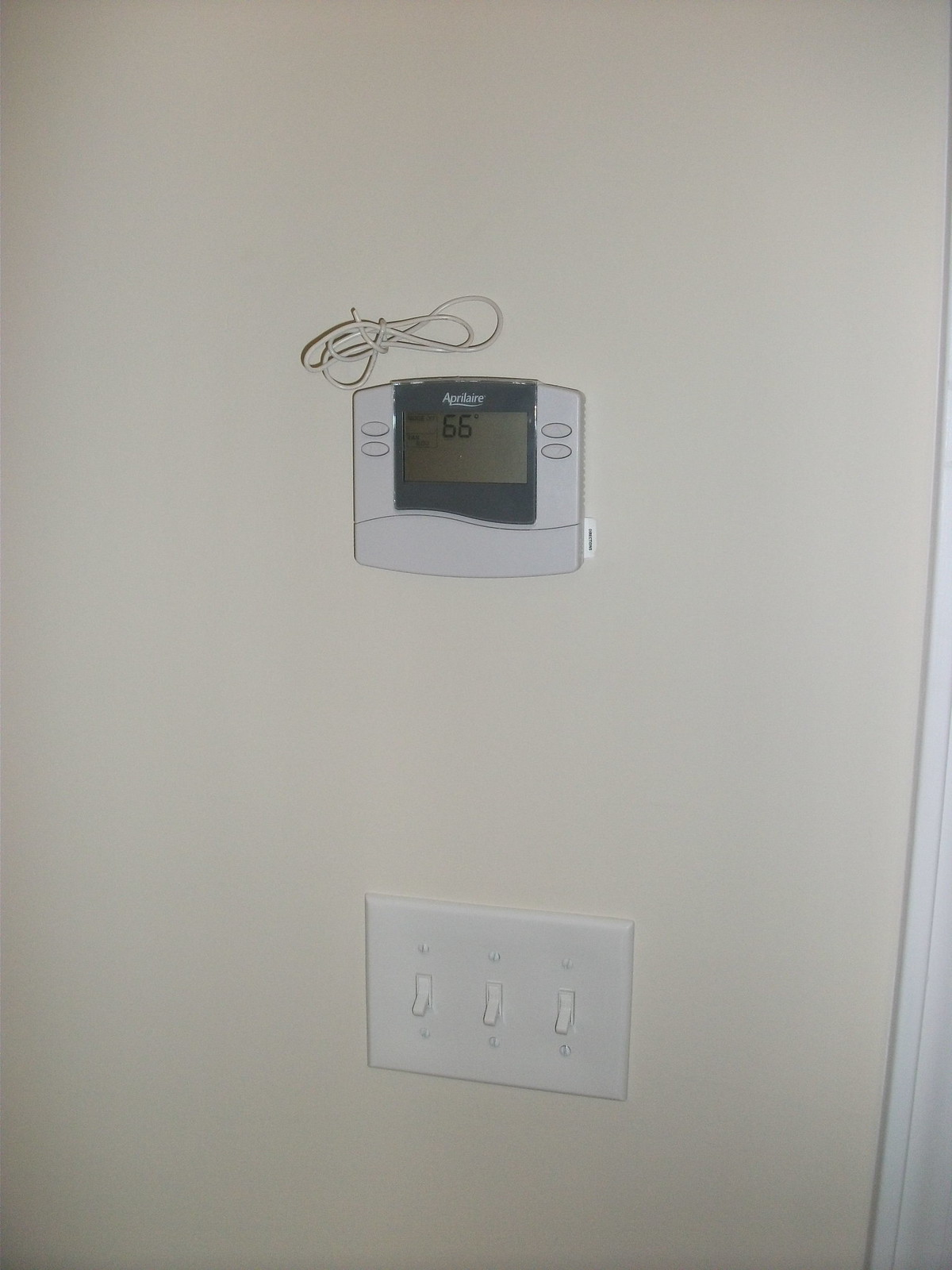The image showcases an interior wall in a building or house, uniformly painted in an eggshell or tan color. On the lower right side of the wall, there is a section of white molding. Positioned at the right center of the wall is an off-white switch plate with three on/off switches, all of which are in the downward (off) position. The switch plate is secured with four screws, two above and two below the switches, which are a slightly darker shade of white at the points where they are turned.

Above the switch plate, there is a modern thermostat featuring a gray and dark-gray color palette. The thermostat's screen displays a logo at the top in white lettering and shows a current temperature of 66 degrees Fahrenheit. The lower part of the screen has some illegible text on the left side. Surrounding the screen are four oval buttons, with two on the left and two on the right. Above the thermostat, a coiled, unused wire extends from the wall, suggesting it may have been set up for a different purpose but is not currently in use.